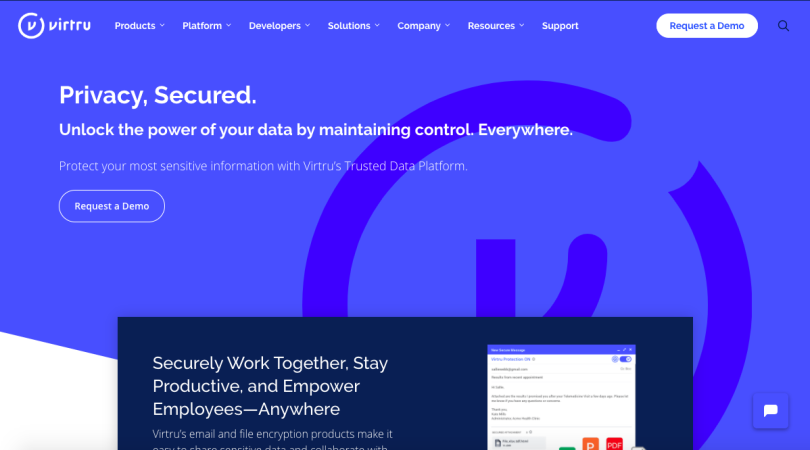This screenshot depicts the main landing page for Virtru, displayed on a blue desktop background. Central to the image is the Virtru logo, consisting of a large, darker blue, broken circle with a 'V' in the middle. Prominent text in the center reads, "Privacy Secured," followed by a smaller subtitle that states, "Unlock the power of your data by maintaining control everywhere." Even smaller text adds, "Protect your most sensitive information with Virtru's trusted data platform," with a "Request a Demo" button situated below.

The bottom portion of the page transitions into a black background with white text that begins to introduce additional features: "Securely work together, stay productive, empower employees." To the right of this text, within the black inset, there's a secondary image that appears to be a screenshot of either a mobile app or another segment of the Virtru application.

At the top of the screen, the website's main menu displays several options: Products, Platform, Developers, Solution, Company, Resources, Support, and another "Request a Demo" button. In the lower right corner, there is a small blue box featuring the universal chat icon, indicating a support or live chat function.